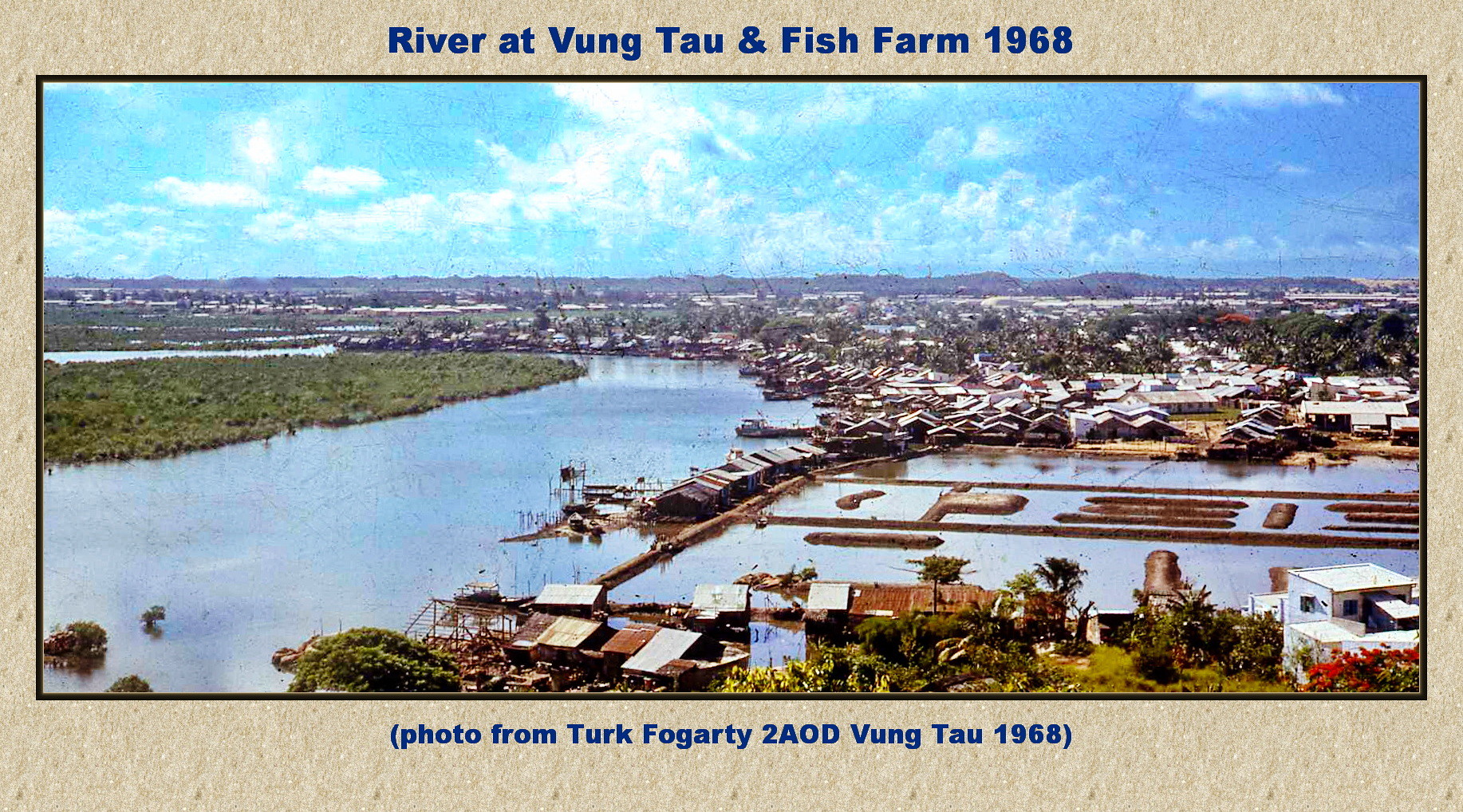This horizontal landscape photograph, shown against a textured, aged white background reminiscent of parchment, is captioned at the top in dark blue print: "River at Vung Tau and Fish Farm, 1968." Below the caption is an aerial view of a winding river that meanders from the lower left of the image towards the center, before bending sharply left again. To the left of the river lies a grassy atoll or island, while the right side features bustling commercial fishing activity, with piers, docks, and fishing stalls. A two-lane channel likely navigated by fishing boats and commercial vessels is visible, flanked by buildings presumed to be unloading docks. In the foreground, a row of buildings lines the mainland's riverbank, giving way to a densely populated village that stretches into the distance on the right side. The background reveals a flat-line mountain range or hillside extending horizontally across the middle of the photograph, beneath a bright blue sky dotted with puffy white clouds. Below the photograph, the same dark blue font is used to provide an additional caption: "(photo from Turk Fogarty, 2 AOD, Vung Tau, 1968)." The entire scene, from the clear skies to the tree-lined riverbanks and summer greenery, captures a vibrant and active riverside settlement in mid-1968.